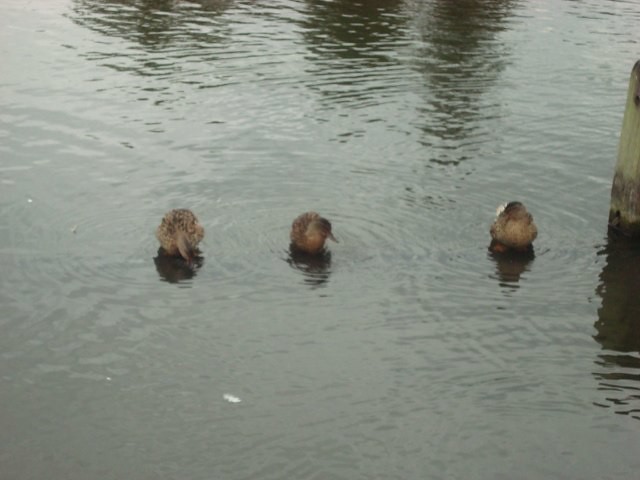This outdoor photograph captures a trio of small, fluffy ducks floating horizontally together on a stretch of dimly lit water, likely a lake or harbour, with grainy quality hinting at overcast daytime conditions. The ducks, evenly spaced and comparable in size, exhibit black and tan feathers with lighter chests. Shadows, possibly from trees, are reflected in the calm, gray water, adding a sense of depth to the scene. To the right, a wooden stake or part of a dock just enters the frame. A white feather, possibly from a seagull, floats about a meter away from the ducks, while the shallow water allows a faint glimpse of their webbed feet.